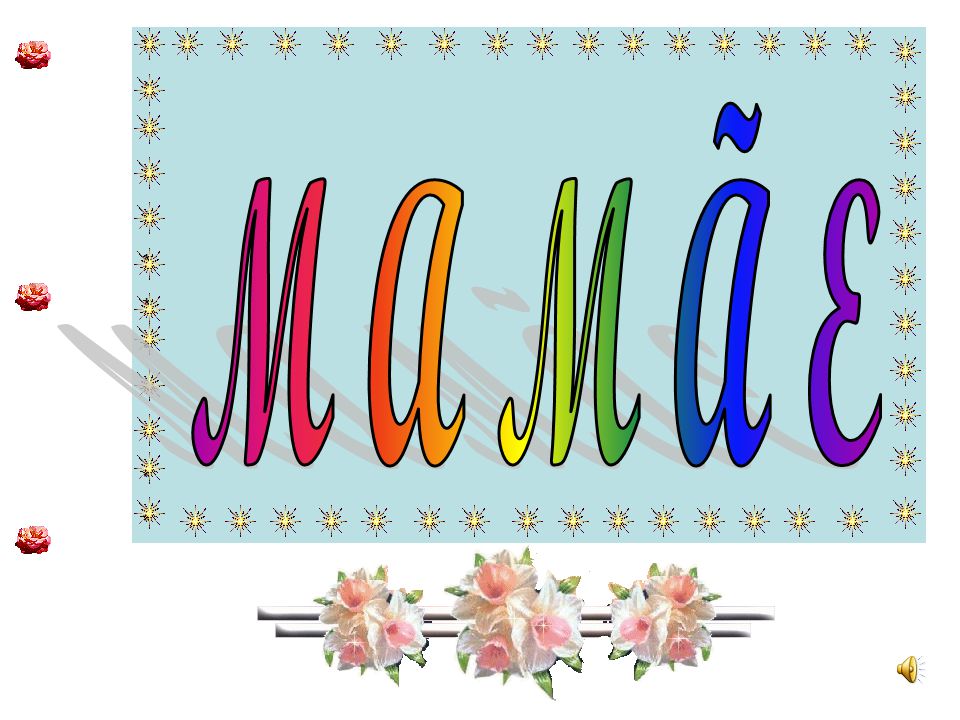The image is a graphic design focusing on a light baby blue rectangular shape, possibly resembling a business card. At the center of the rectangle, the text “MAMÃE” appears in large, multicolored letters, each letter transitioning from purple to red to dark orange, orange, yellow, green, dark green, blue, and purple, with a noticeable drop shadow extending towards the top left. Surrounding the light blue rectangle is a border formed by starburst shapes, creating a dynamic frame.

In the bottom central part of the image, there are three pink and white flower illustrations arranged in bouquets, with green leaves, connected by two simple silver bars that appear like computer graphics or WordArt. These bouquets add a delicate touch to the otherwise vibrant design.

To the lower right corner, a yellow interactive-looking speaker icon suggests an audio component, while along the left side of the blue rectangle, three small rose icons are dotted vertically from top to bottom.

Overall, the image emits a crude yet colorful aesthetic, blending multiple graphic elements into a cohesive and eye-catching design.